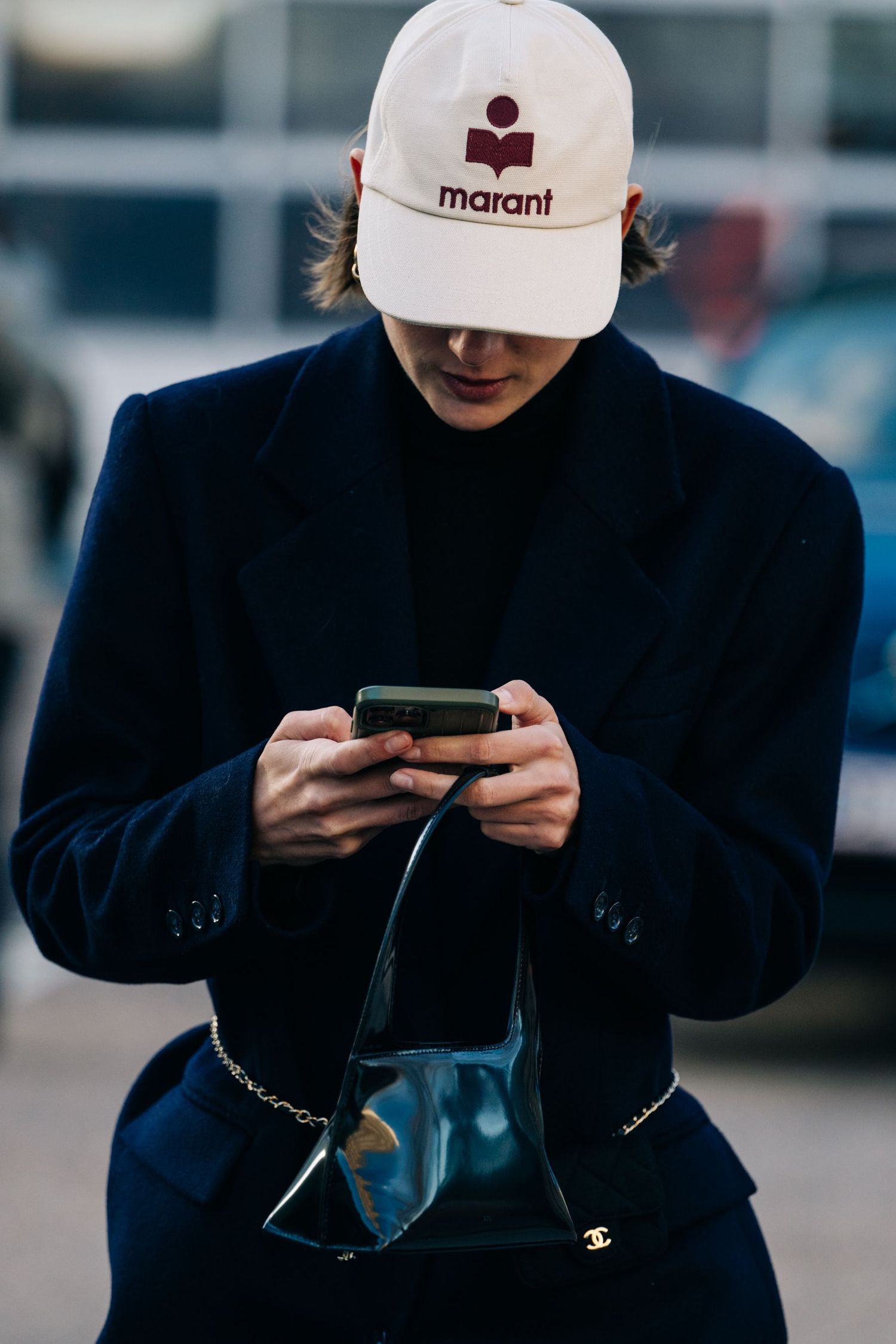The photograph features a Caucasian woman, illustrated with an emphasis on her stylish attire and accessories. She is sporting a navy blue, long peacoat adorned with distinctive big blue buttons on its sleeves. Accompanying this is a white baseball cap bearing the maroon logo and text 'Marant'. The cap strategically shades her face, partially concealing her features and revealing just her nose and mouth, which are complemented by dark red lipstick. Her shoulder-length, light brunette hair is tucked neatly behind her ears beneath the cap. The woman clutches a modern Android cell phone encased in a green cover with both hands, fixating her gaze downward towards the device. Additionally, she carries a small, shiny black Gucci handbag made of leather. The background captures a blurry scene, possibly depicting a car, a road, and maybe a building or a white garage with black windows, indicating an outdoor setting likely during late afternoon.